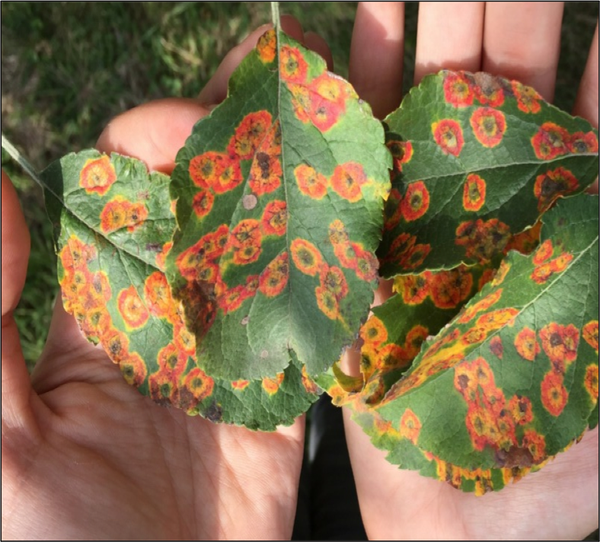The image is a square-shaped, outdoor photograph taken during the daytime, framed by a thin black pinstripe border. We are looking down at a Caucasian man's hands, positioned with their palms up and side by side over a bed of green grass. His left hand appears on the left side of the image, partially in shadow, with its thumb visible and fingers emerging from the bottom, the wrist not fully within view. His right hand is on the right side of the image, well lit by sunlight, with fingers extending slightly out of the frame. Within his hands, he holds several elliptical green leaves, each adorned with intricate orange and yellow oval patterns, possibly indicative of a plant disease. These designs feature dark central dots, creating a striking contrast against the vibrant green of the leaves. The patterns are more concentrated on some leaves than others, hinting at variation in the severity of the spotting. Additionally, the man's left foot, clad in a shoe, is partially visible in the grass near his left hand.